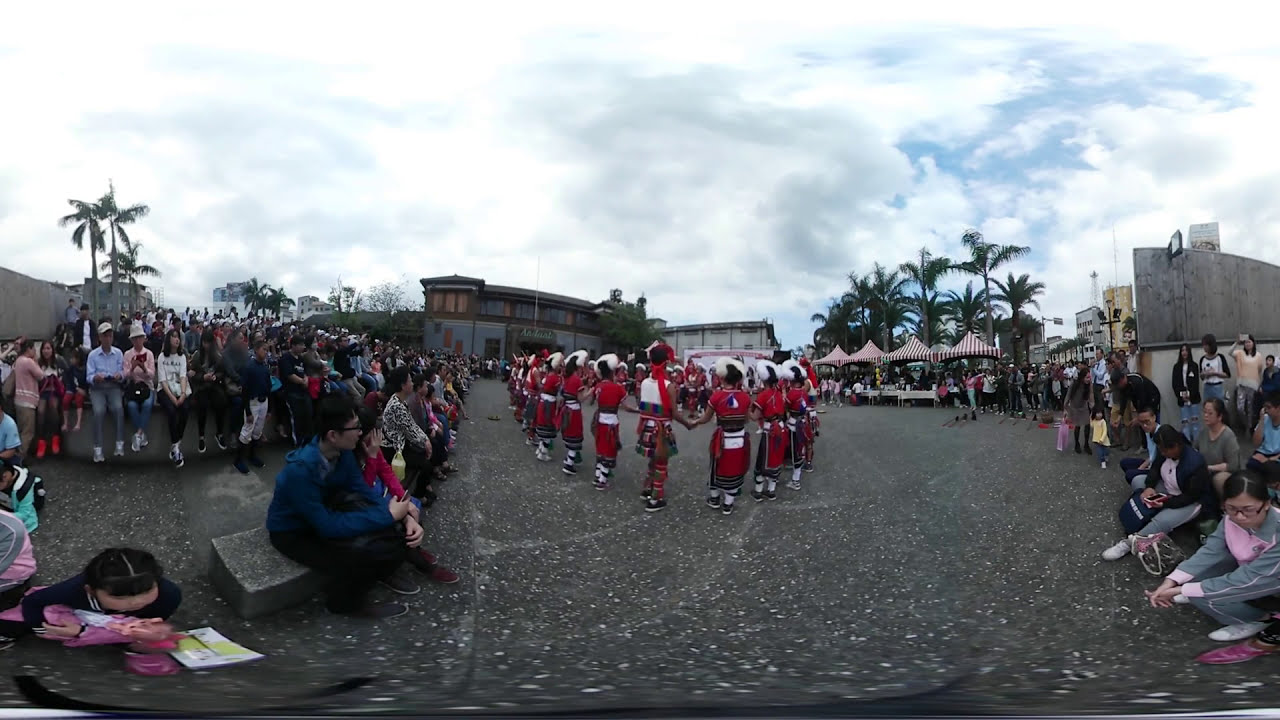A large group of people are gathered at an outdoor event, possibly a ceremony or dance performance, taking place on a black asphalt ground speckled with white. At the center, a circle of individuals, all with black hair and dressed in red outfits adorned with white feathered head dressings, hold hands. One person among them has a distinctive white patch on their back. Surrounding this circle, spectators are seated on various types of benches. To the right, a woman in a gray jacket with pink accents and glasses looks downwards, appearing somewhat disinterested. On the far left, a girl with long black hair, parted in the middle and extending below her back, also gazes downwards. She wears a pink outfit and has a yellow and white paper in front of her. Next to her, a man in a blue shirt and black pants, with crossed legs and arms resting on his shins, watches on, though his expression isn't fully engaged either.

The background reveals an urban landscape with a mix of buildings. To the right stands a gray-walled building with an arched top, alongside a yellow-colored structure and a shorter gray building with a radio antenna. A group of palm trees is visible, flanked by canopies with red and white stripes. Other buildings in light gray and orange hues add to the cityscape. Above these structures, a mostly cloudy sky with glimpses of blue on the right provides a vivid backdrop.

The setting suggests a festive yet somewhat subdued atmosphere, with tents potentially offering souvenirs and refreshments. The overall scene conveys a mix of cultural richness and casual disinterest from the audience, capturing the event's ambiance under a partly sunny sky.